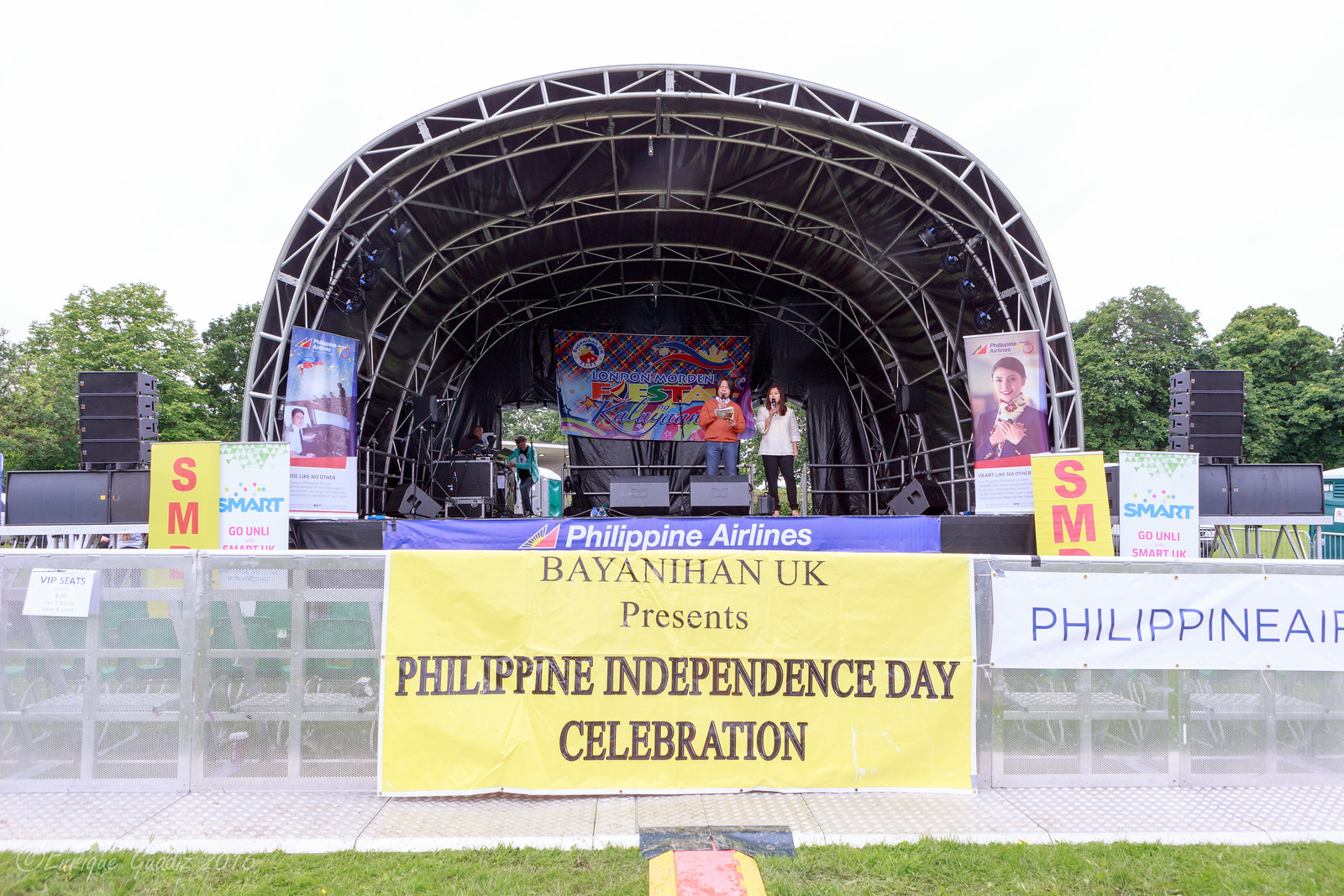In this detailed image set outdoors in the middle of the day, the foreground features a patch of green grass alongside a sidewalk. The scene is framed by a fence-like divider with various signs, including a prominent banner that reads, "Philippine Airlines, BAYANIHAN UK presents Philippine Independence Day Celebration." At the center stage, partially covered by a semicircle canopy, stand two people holding microphones, poised to address the audience. Flanking the stage on both sides are additional signs and equipment on tables. In the background, a serene array of green trees stretches beneath a clear sky. The vivid colors in the image include green, yellow, pink, tan, black, blue, red, gray, and purple, adding vibrancy to the festive atmosphere celebrating Philippine Independence Day.